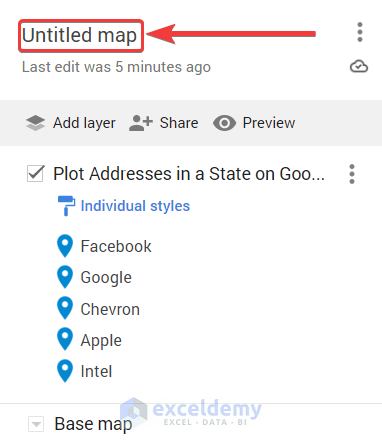The image displays an untitled map interface with various navigation and editing tools:

1. At the top, there's a title labeled "Untitled Map," highlighted with a red box and indicated by a red arrow.
2. On the right side, a vertical ellipsis is present above a cloud icon.
3. Beneath the red box, the text reads "Gray Text, last edit was five minutes ago."
4. Below this, a gray box features a square icon accompanied by the text "Add Layer."
5. Adjacent to it is an icon of a person with a plus sign, labeled "Share." Nearby, an eyeball icon marked "Preview" is visible.
6. A box with a check mark states "Plot Address is in a State on Google," with a vertical ellipsis to its right.
7. Further down, a blue rolling paintbrush icon labeled "Individual Styles" is shown.
8. Five company names—Facebook, Google, Chevron, Apple, Intel—each have a blue location pin beside them.
9. At the bottom, the text "Base Map" is followed by "Sell to Me Excel Data."

This detailed view provides a comprehensive overview of the map interface elements, their functions, and the associated data points involved.